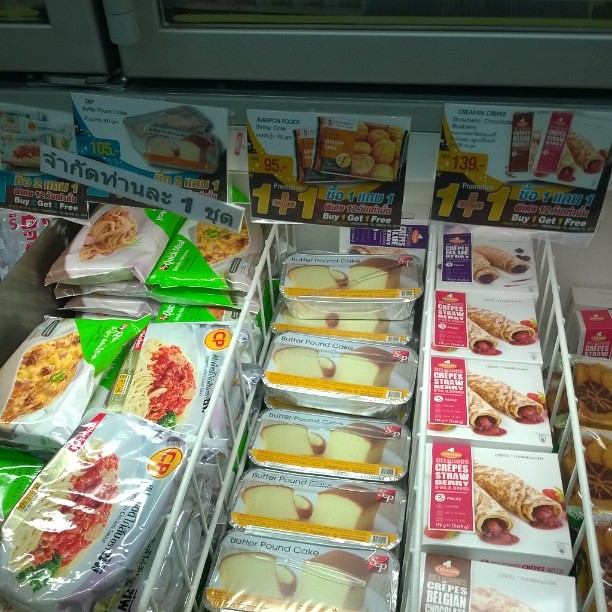The image showcases a vibrant selection of ready-to-eat and frozen meals within a waist-level freezer section, most likely in a convenience store or frozen food market. The rectangular section is neatly divided by white bars, organizing an array of appetizing items. Prominently visible is a Butter Pound Cake in a rectangular tin, with a clear label on the packaging. Nearby, there are various crepes, including strawberry and berry flavors, displayed alongside other enticing frozen desserts. Off to the left, a sign featuring unfamiliar characters, possibly Middle Eastern, flanks the display with prominent, multilingual pricing. The scene is an inviting snapshot of diverse, convenient culinary delights.